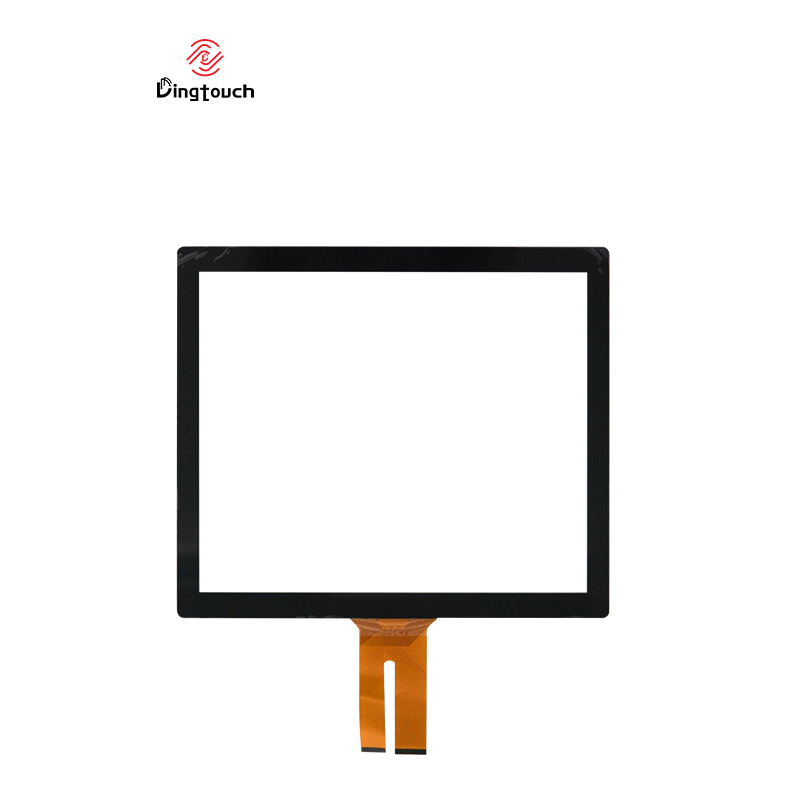The image features a white background with a centrally positioned square that has a solid white interior and a thick black border, reminiscent of a blank screen. Extending down from the middle bottom edge of the square are what appear to be two orange, rectangular shapes resembling cartoonish legs with black borders at the bottom, possibly representing shoes. These "legs" are speculated to support the square. In the top left corner of the image, there is text reading "DingTouch" in black letters below an intricate red eye-like logo with swirling lines, giving the impression of the center of a tornado. The overall composition suggests a promotional photograph of a product named DingTouch.